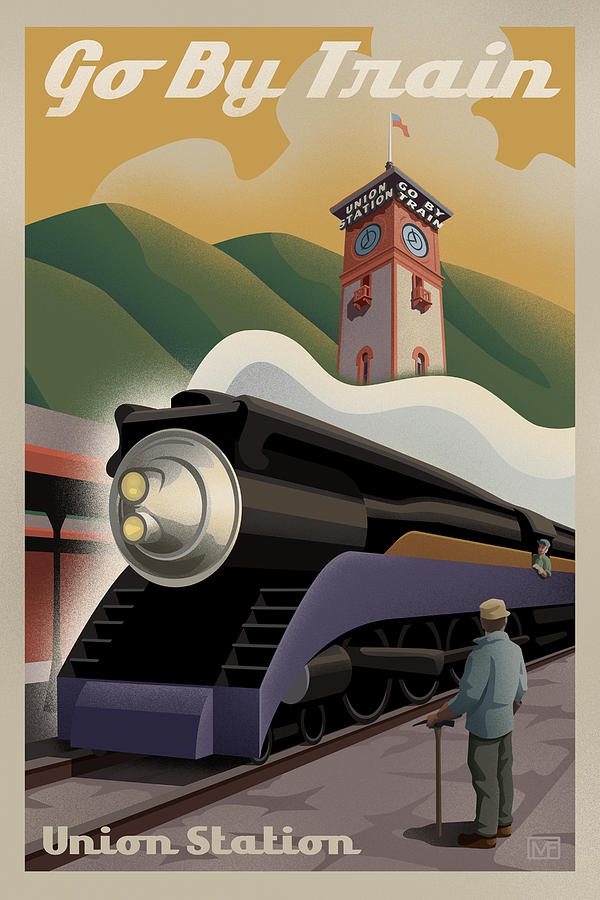The promotional poster features an illustrated scene of Union Station with a strikingly vintage aesthetic. Dominating the top of the image is an orange-hued sky with patches of white clouds and the bold off-white text “Go by Train.” Below, verdant green hills with yellow highlights create a picturesque backdrop for the central elements of the poster. 

In the middle of the image stands a prominent clock tower adorned with an American flag at its peak, with "Union Station" and "Go by Train" emblazoned on its red-hued structure. The clock on each side of the tower features a blue face. Below the tower, a sleek train is depicted as it heads into the station. The train itself is purple on the lower half with a gold stripe, transitioning to a black main engine compartment with a silver front. White smoke billows out, further enhancing the nostalgic feel.

In the foreground, a man stands waiting for the train. He is dressed in green pants, a blue jacket, and a tan hat, and he is leaning on a cane. The entire image is bordered by a tan-colored frame, and in the bottom right-hand corner rests a watermark featuring an "M" with an "F" inside a rectangular box. Additionally, the bottom left corner of the image contains the words “Union Station” in the same off-white text as above.